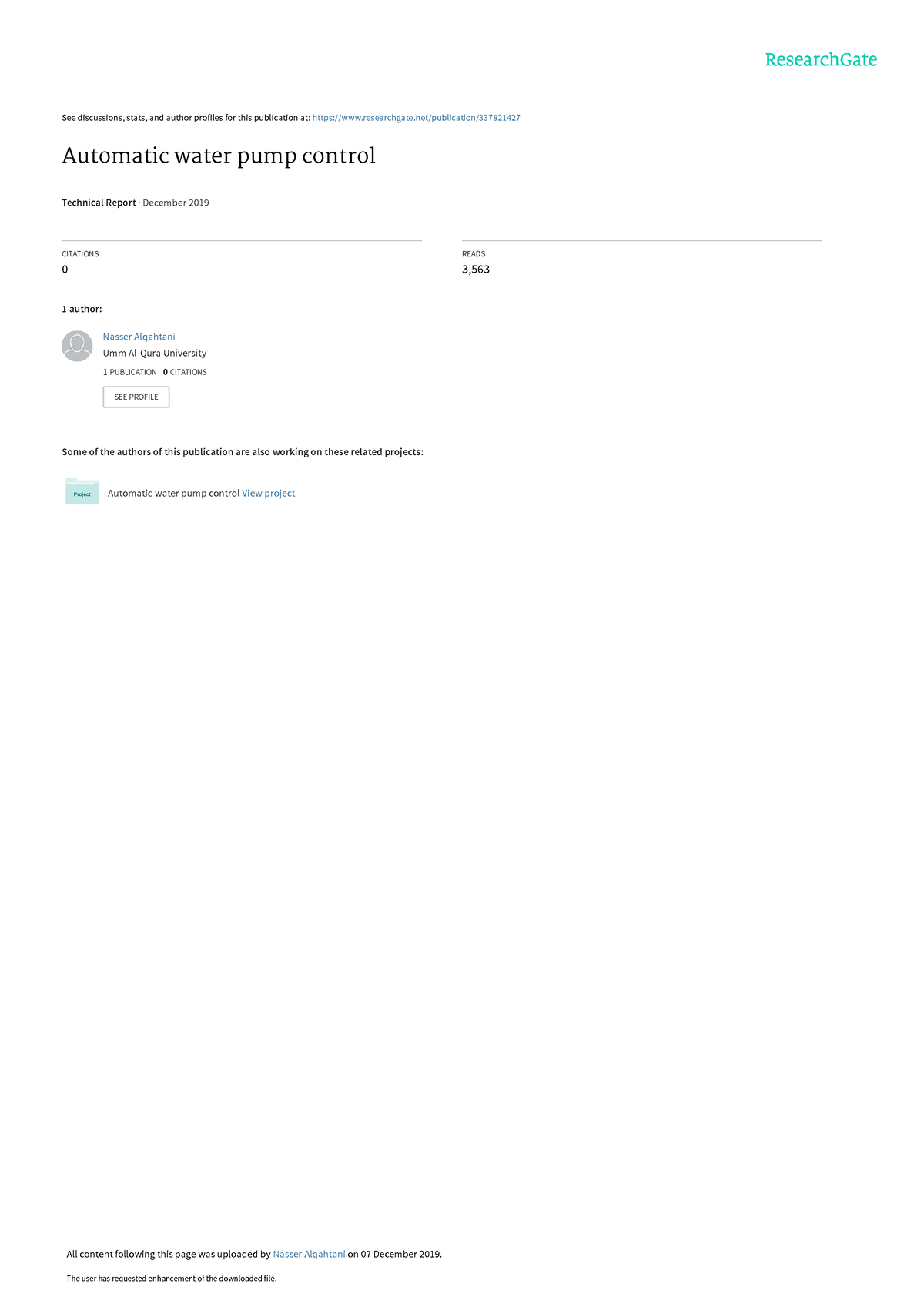This image is a detailed excerpt from a document, likely sourced from the ResearchGate website. The document features a predominantly white background with black text. In the top-right corner, prominently displayed, is the ResearchGate logo, featuring the word "ResearchGate" as one word with both 'R' and 'G' capitalized, and is styled in a teal, greenish-blue color.

On the upper-left side of the document, there is a small text section that reads: "See discussions, stats, and author profiles for this publication," followed by a hyperlink to the ResearchGate website (researchgate.net), along with the specific publication number. 

Beneath this, the title of the document is stated as "Automatic Water Pump Control," accompanied by the designation "Technical Report." It also indicates that the report was published in December 2019. Additionally, it provides statistics, noting "0 citations," "3,563 reads," and lists "1 author." The sole author is named Nasir Alqahtani, affiliated with Umm Alqahtani University, and it is noted that this is his only publication.

The overall layout of the document is clean and primarily textual, aimed at presenting a concise summary of the publication's essential details.